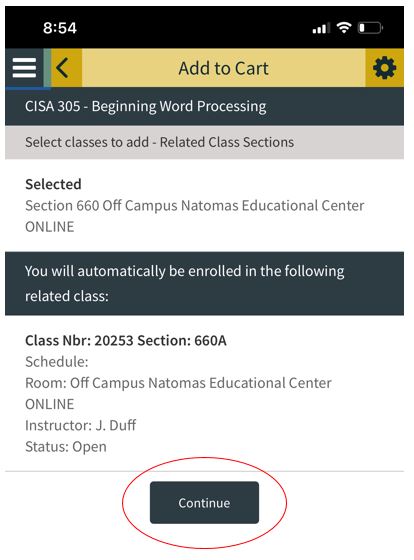Screenshot displaying a mobile interface with detailed elements:

At the top of the phone screen, there is a distinctive black bar with a current time displayed as 8:54, although it's unclear if it's AM or PM. The signal strength is indicated by three bars, and the battery icon shows critically low battery life.

Below this bar, there is a hamburger menu icon next to an 'Add to Cart' button within a text input field, characterized by a tan color. To the right of this, there is a brownish-orange back arrow and a similar colored settings gear icon. Under these icons, the text reads "CSC is a" followed by "305" indicating the start of a word processing session, highlighting various options available for adding to the cart.

Further down, the text instructs to "Select classes to add," suggesting that the user is enrolling in classes, showing potential class sections to choose from. The section "Selected Section 660" is highlighted, with details indicating it's an off-campus course at the Natomas Education Center and available online. 

Additional information includes an automatic enrollment notice for related classes, specifying class NBR 20253 under section 660, scheduled at the off-campus Natomas Educational Center with instructor J. Duff, and marked as open for registration. 

The interface concludes with a prominent red 'Continue' button at the bottom of the screen, encouraging the user to proceed with their selection.